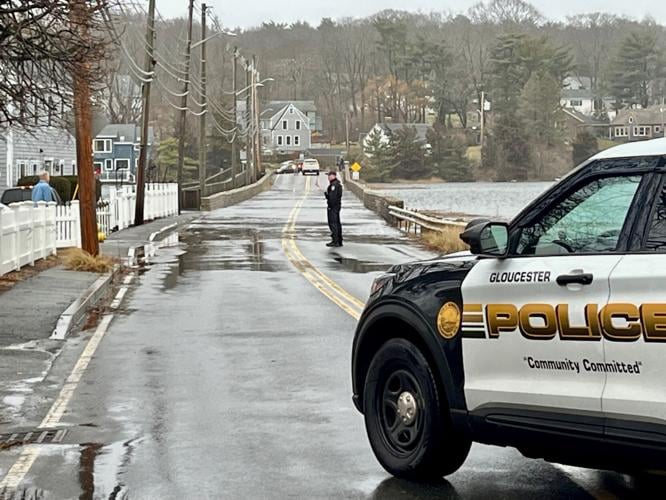In this color photograph, we see a wet, rain-soaked street in a residential area, closed off by police vehicles. Central to the image is a white and blue police car with gold lettering that reads "Cloutchester Police" along the side, and the slogan "Community Committed." The vehicle is positioned in the middle of the road, blocking traffic in both directions. The scene features a policeman approximately 100 feet down the road, standing near the middle and seemingly in conversation with a bystander who lives in one of the houses aligning the street. 

On the right-hand side of the image, closer to the foreground, only the front end of the police car is visible. A secondary police vehicle appears further down, blocking the opposite end of the road. Along the left, there is a white picket fence with a man standing inside his yard, typical of this suburban environment. The street is lined with utility poles and streetlights, with houses stretching towards the background. In the background, there are leafless trees and a field with patches of melting snow, suggesting it is winter. A body of water is visible behind the police car in the upper right-hand side, completing this tranquil yet cordoned-off streetscape.